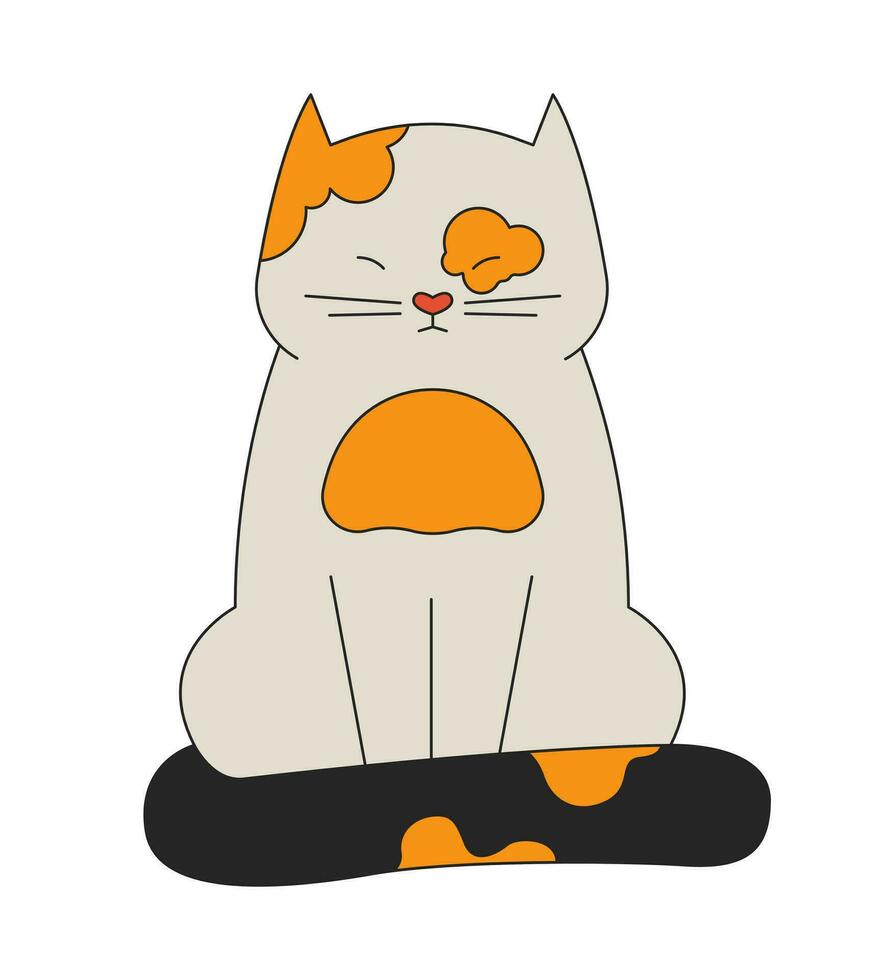This digital cartoon-style illustration features a plump, white cat sitting and facing the viewer with an expression reminiscent of traditional Asian art due to its slit-like eyes. The cat has a distinctive heart-shaped, dark orange nose, four whiskers (two on each side), and a content, almost serene expression. Notably, it sports various orange splotches: one on its left ear, one around its right eye, and a larger one on its chest. Its black tail, which wraps around its front legs, also displays two orange splotches. The inconsistencies in the cat's coloring and its tranquil pose make it a charming and unique depiction.